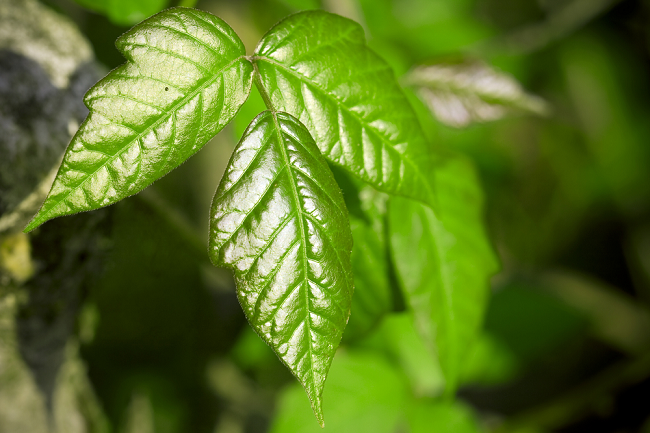This detailed close-up photograph features a trio of medium-sized, pointed leaves, arranged in a triangular formation on a single stem. The leaves, exhibiting parallel veins, have a smooth, shiny texture that reflects light, suggesting a well-lit environment. Each leaf, showcasing a combination of light and dark green hues, with one displaying a hint of red, has slightly jagged edges. The background reveals a blurred canvas of additional green foliage, interspersed with indistinct shapes in shades of black, gray, and brown, which could potentially be rocks or pots. This focus on the vibrant, meticulously detailed leaves renders the surrounding environment indistinguishable, highlighting the nuanced beauty of the leaves themselves.